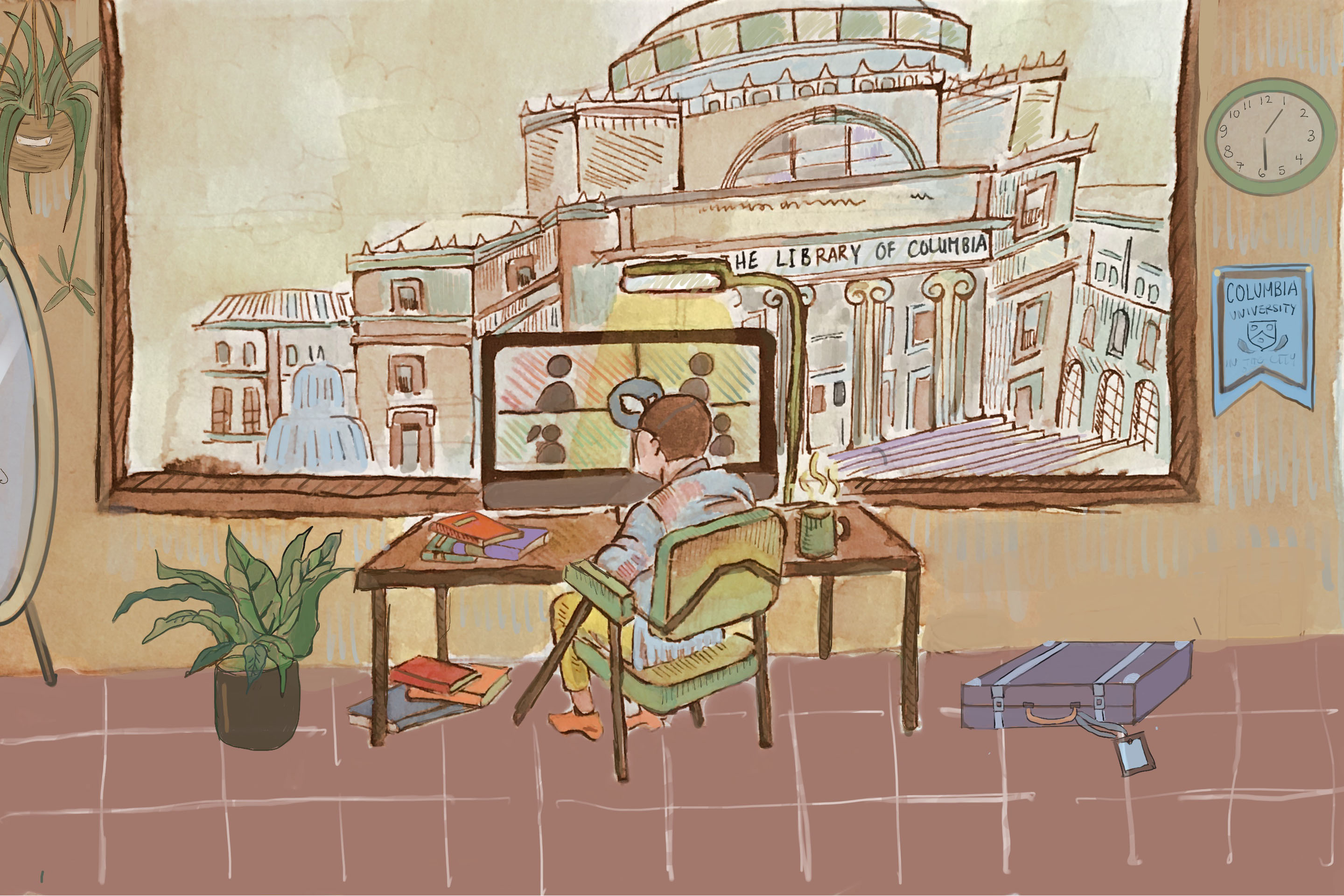In a detailed cartoon-like painting, a human figure is seated in a green chair facing away from the viewer, immersed in a computer screen on a wooden desk. The person, who has short brown hair, light skin, wears yellow pants, and orange shoes, is surrounded by various items. To the person's left, a potted plant adds a touch of greenery, while a green mug with visible steam sits to their right, suggesting a freshly brewed beverage. On the desk, three books are stacked; a red book on top, followed by a purple one, and a green one at the bottom. Additional clutter includes three books on the floor under the desk – red, orange, and blue – and a blue suitcase to the right of the chair.

The scene is set in what appears to be an office or study, illuminated by an overhead light. The back of the room features a large window or portrait that occupies almost half the image, revealing a view of the grand Library of Columbia building, adorned with the words "Library of Columbia." The backdrop includes extra details like a banner for Columbia University, a green and white clock above it, and in the far-left corner, a mirror hangs beside hanging plants. The painting captures a serene yet busy atmosphere, with the man possibly engaged in a Zoom meeting, as he works at his desk.